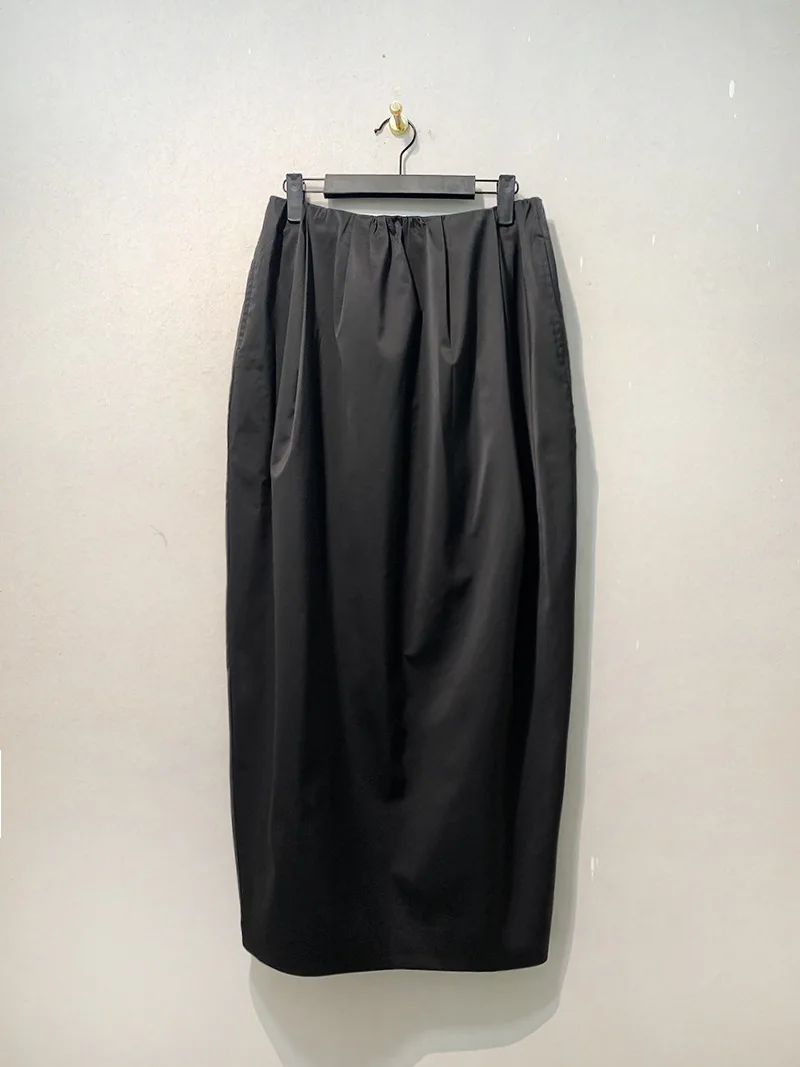In this image, a black pencil skirt is prominently displayed against a blank gray wall, creating a minimalist and focused composition. The skirt is hanging from a specialized black skirt hanger, which features a wire hook and a central stabilizing horizontal bar, possibly made of wood or high-quality plastic. This hanger is attached to a beige peg protruding from the wall. The hook of the hanger secures itself to this peg, which somewhat resembles a small door stopper in appearance. The skirt itself is smooth and appears well-maintained, with only slight creases suggesting it is well-fitted and possibly tailored. There are no visible buttons, zippers, or other fasteners, indicating it may have a simple design with possibly a bit of elastic for fit. The skirt casts a subtle shadow on the wall, contributing to the overall clean and uncluttered aesthetic of the image.